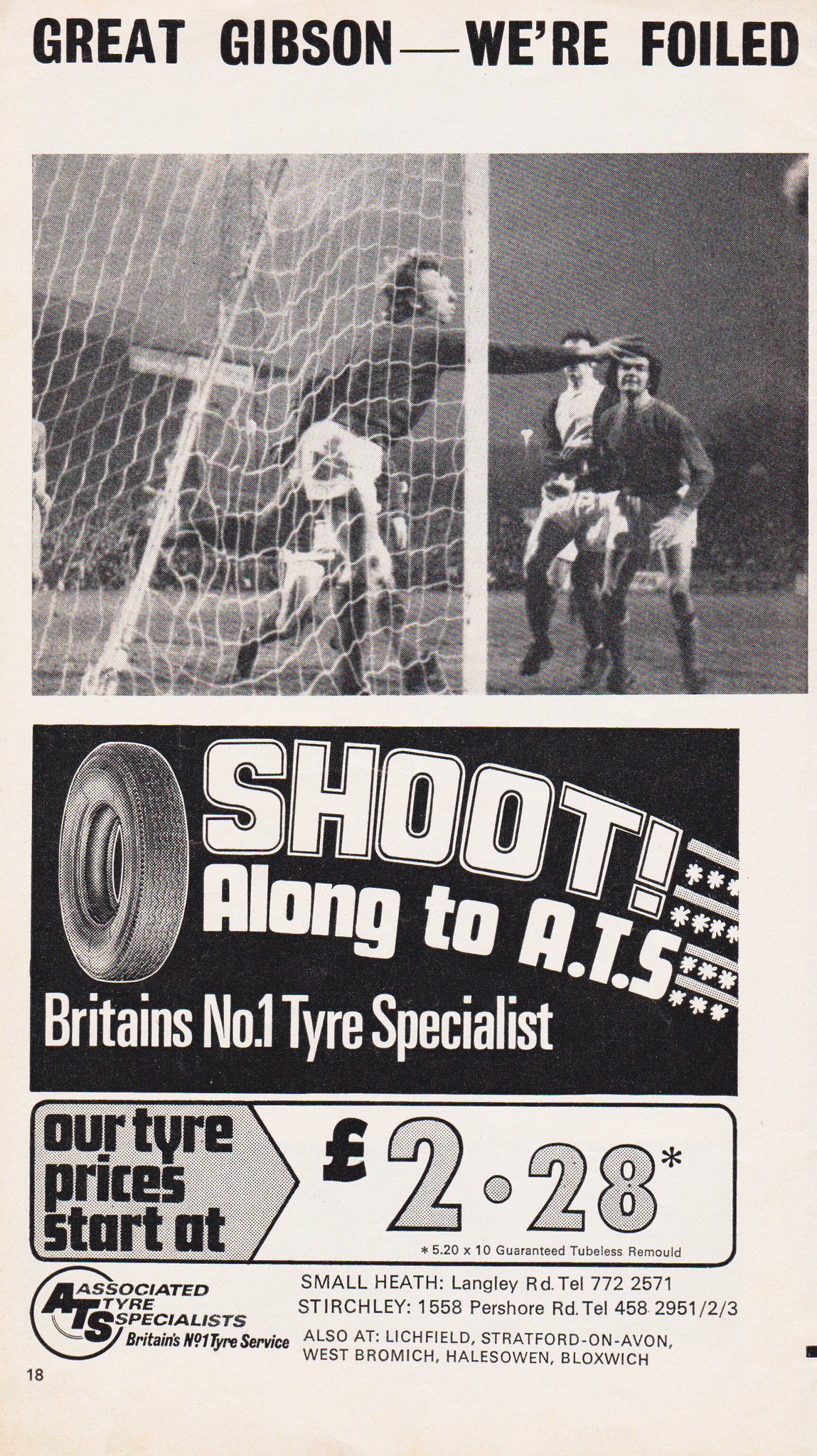The image depicts a page from an old magazine with a light gray, off-white background. At the top, bold black text reads "Great Gibson - FOILED." Below this headline, a black and white photograph captures an intense moment on a soccer field. The central focus is a goalie dressed in a dark, long-sleeved shirt and shorts featuring black and white designs. The goalie’s hand is reaching above a player in a dark shirt with white shorts, attempting to intercept the ball that is descending from the upper right corner. Adjacent to the goalie on the right, another player dressed in a white shirt and white shorts is rushing towards the ball. The soccer goal features a prominent white round bar up the center, supporting the net behind which the goalie is visible.

The bottom half of the page is dedicated to advertisements. The initial ad is set against a black background, with a tire image and bold text proclaiming "SHOOT!" followed by "along to A.T.S. Britain's number one tire specialist." Below this, another rectangle highlights, "Our tire prices start at £2.28," accompanied by the name "Associated Tire Specialists" and various addresses and telephone numbers. The number 18 is indicated in the bottom left corner, possibly denoting the page number. The vintage feel is accentuated by the dated tire prices and black-and-white print, suggesting that this magazine page is from a bygone era.